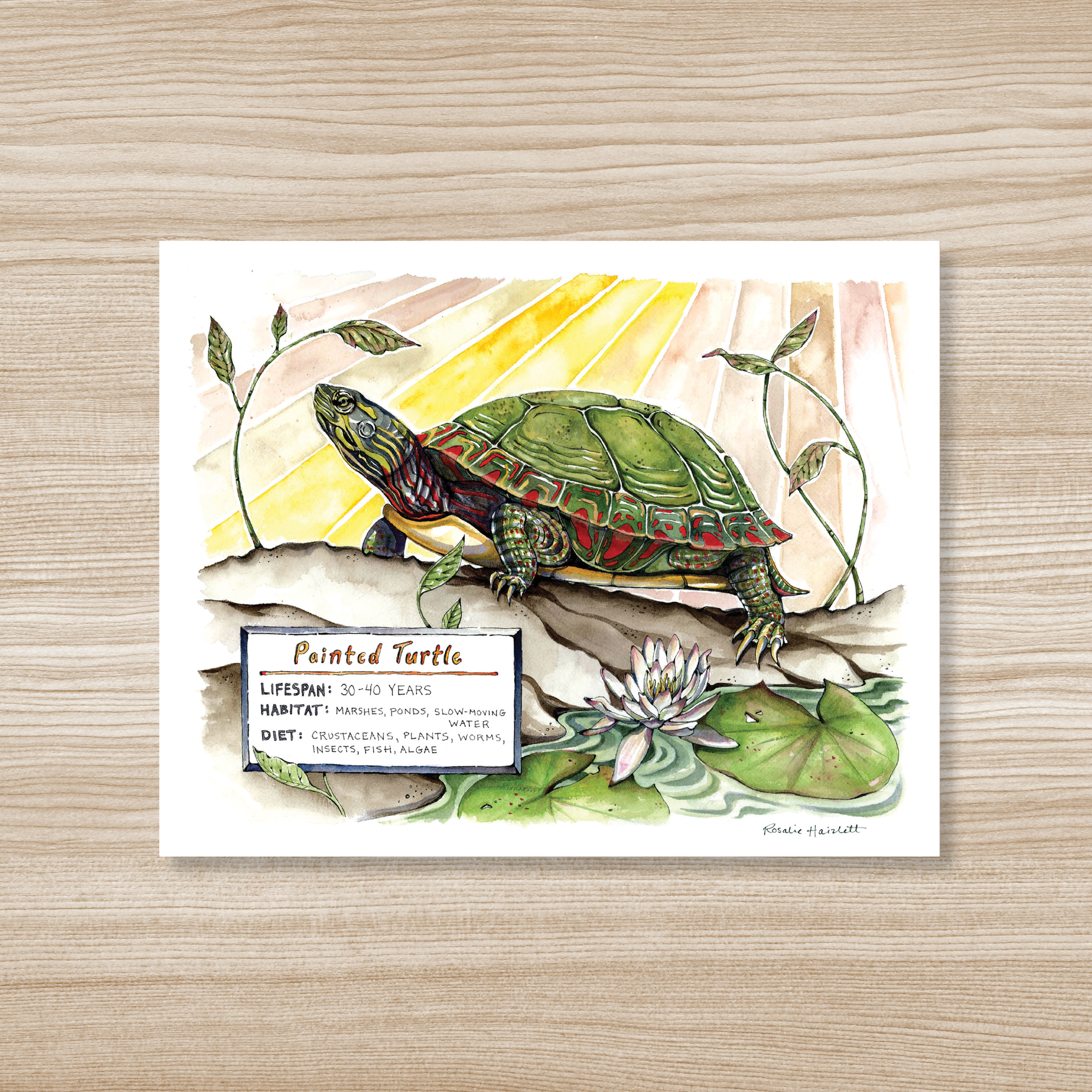This detailed illustration by Rosalie Harlett on white paper, set against a light-toned wood grain surface, showcases a painted turtle in vibrant watercolors. At the center, the turtle, adorned with green and red hues, is climbing on land with its head positioned to the left, displaying distinct stripes on its head and neck. Its body partially conceals the back right leg, while the other three legs and its big claws are visible. The turtle's environment is rich with detail, featuring a nearby water body with lily pads and a white blossom underneath its left leg. To the left and right of its head are sprouts with three leaves each. The background is adorned with rays of sunlight in pink, orange, and light brown tones, adding warmth to the scene. In the bottom left corner, an informative box details the painted turtle’s lifespan of 30 to 40 years, its habitat in marshes, ponds, and slow-moving water, and its diet of crustaceans, plants, worms, insects, fish, and algae. The bottom right corner bears the signature of the artist, Rosalie Harlett.